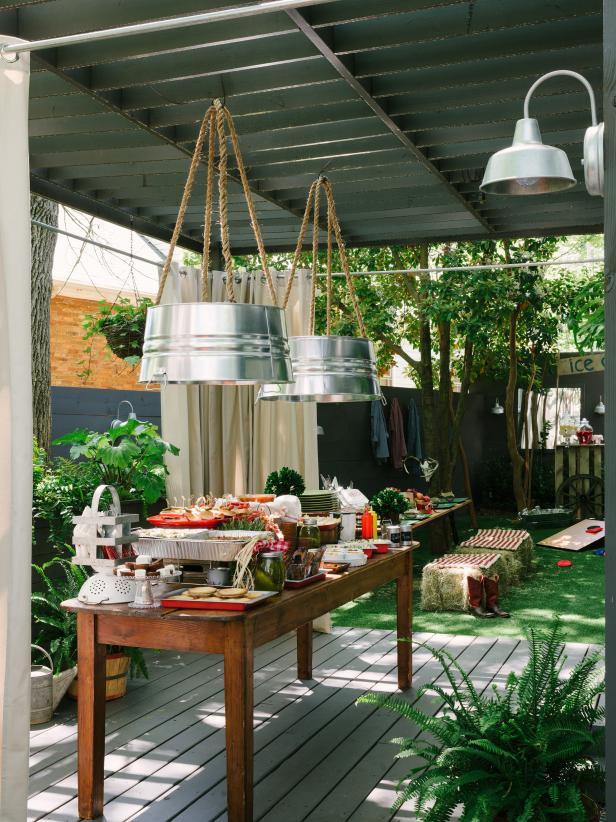This is a photograph of a lively outdoor party on a wooden deck in a fenced backyard. The deck, painted in shades of gray and black, features a long wooden table adorned with a variety of food items, some of which are served in raised tin trays likely kept warm underneath. Plates are visible at one end of the table. The yard is decorated with numerous large leafy green plants and potted greens. Makeshift lights created from buckets turned upside down and hung by ropes illuminate the scene. A pair of hay bales with cloth coverings serves as makeshift seating, next to which a pair of cowboy boots can be spotted. The party appears crowded, with additional details like shirts hung on the fence and outdoor games such as cornhole set up on the grassy area. The sun is shining brightly, enhancing the festive atmosphere of the gathering with a neighbor's brick house visible in the background.